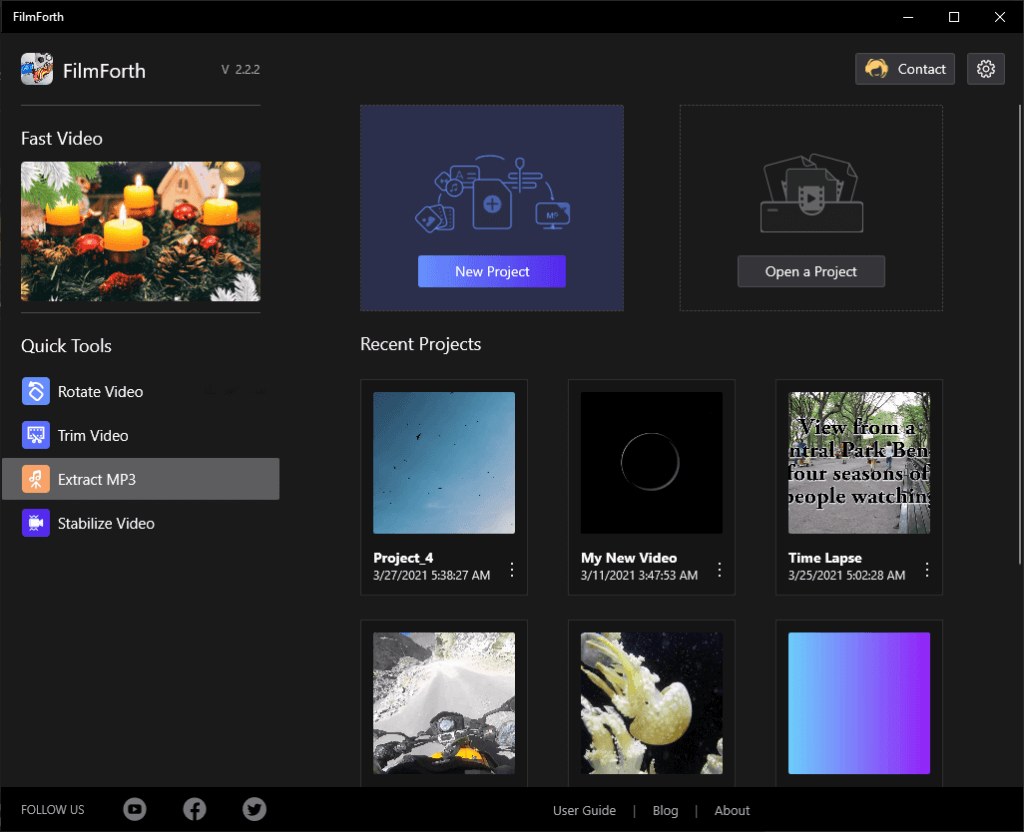This screenshot from Filmforth (spelled F-I-L-M-F-O-R-T-H) captures the interface of version 2.2.2 of the software. At the top of the screen, there's a header displaying "Filmforth V 2.2.2" alongside options for "Contact" and a gear icon for settings. 

On the left, there's a vertical menu listing several options: "Fast Video," complemented by an image showcasing a festive Christmas table setting adorned with pine boughs, lit pillar candles, a small white house sculpture, and various Christmas ornaments. The menu continues with options for "Quick Tools," including "Rotate Video," "Trim Video," "Extract MP3" (which is currently selected), and "Stabilize Video."

The right side of the screen features multiple screenshots arranged vertically. At the top, it lists options for "New Project," "Open a Project," and "Recent Projects." Below, a project titled "Project 4" dated 3-27-2021 at 5:38:27 AM displays an image of a blue sky dotted with dark specks. Next is "My New Video," with a date of 3-11-2021 at 3:47:53 AM, displaying a black square with a white circle in the center. Following is "Time-lapse," dated 3-25-2021 at 5:02:28 AM, showing a photograph of a park with a title that reads, "View from a Central Park Bench, Four Seasons of People Watching."

Continuing downward, the writing cuts off, but the visible section shows an image from the rider's point of view on a motorcycle, cruising down a desert highway. There’s another image showcasing pale yellow jellyfish floating downward, followed by a gradient square transitioning from blue on the left to purple on the right.

At the bottom of the right section, there are additional options labeled "User Guide," "Blog," and "About."